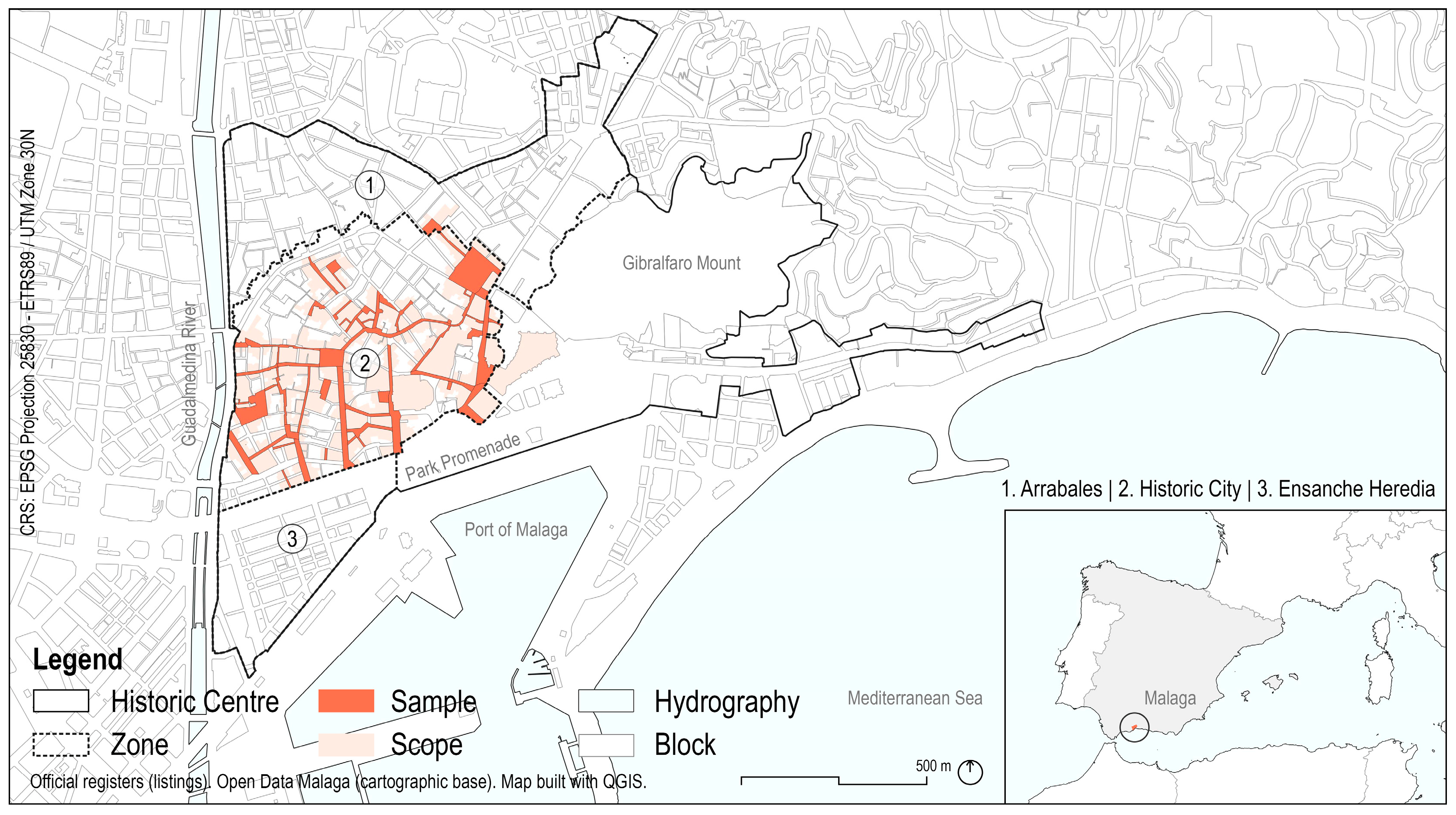The image is a detailed, professionally drawn map of the city of Malaga, Spain, with a focus on its historic center and surrounding areas. The map is predominantly black and white, with key features and zones highlighted in color. A legend at the bottom of the map explains that "historic center" and "zone" are depicted in white, "sample" is in deep orange, "scope" is in light pastel pink, and "hydrography" (water bodies) is shown in light blue. The legend also includes categories such as "block". 

The map is outlined in black and includes various labels and features: CRS EPSG Projection 25830 ETRS89 UTM Zone 30N is noted at the top left corner. Important locations such as the Port of Malaga, Park Promenade, Gibralfaro Mount, and the Guadalmedina River are clearly marked. At the bottom right, there's a boxed-off section that highlights different areas within the city, labeled as 1 Arraiales, 2 Historic City, and 3 Ensanche Heredia, all shaded in gray.

The streets on the map are marked with various lines, indicating roads and pathways, and the Mediterranean Sea is shown in light blue at the bottom. A smaller inset map in the bottom right shows a broader view, possibly including parts of Spain, Portugal, and North Africa, pinpointing Malaga with a circle and dot.

Overall, the map is a comprehensive cartographic base of Malaga, created with QGIS and sourced from official registers and open data.